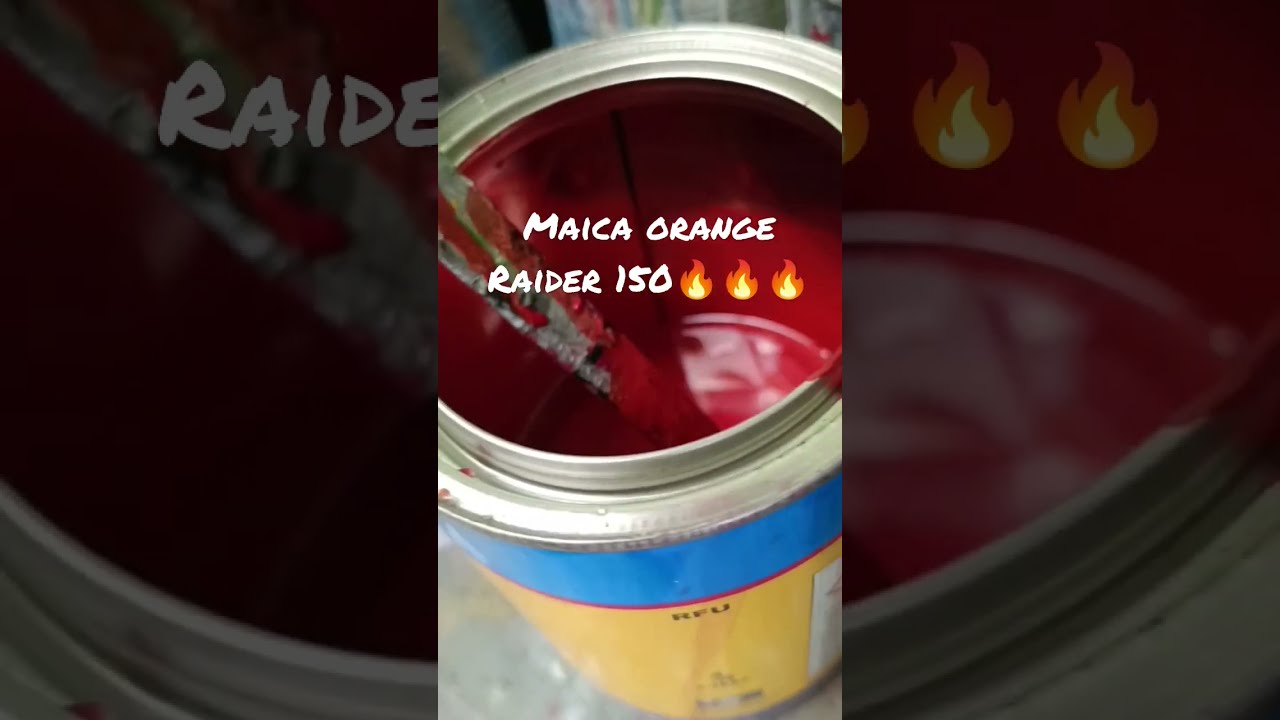The image depicts a high-quality, color photograph centered around a paint can filled with vivid red paint. The can features text slightly above the middle point that reads "Mica Orange Raider 150" in white letters, accompanied by three flame emojis, illustrating a fiery, intense theme. The paint can is the sole object in the image, and it's enveloped in abundant natural daylight, suggesting a daytime setting. The image composition includes framed elements on the left and right sides, which appear to be fragmented reflections of the central scene, contributing to a layered visual effect. The overall imagery is clear and well-lit, though there are no people present, emphasizing the focus on the paint can itself.